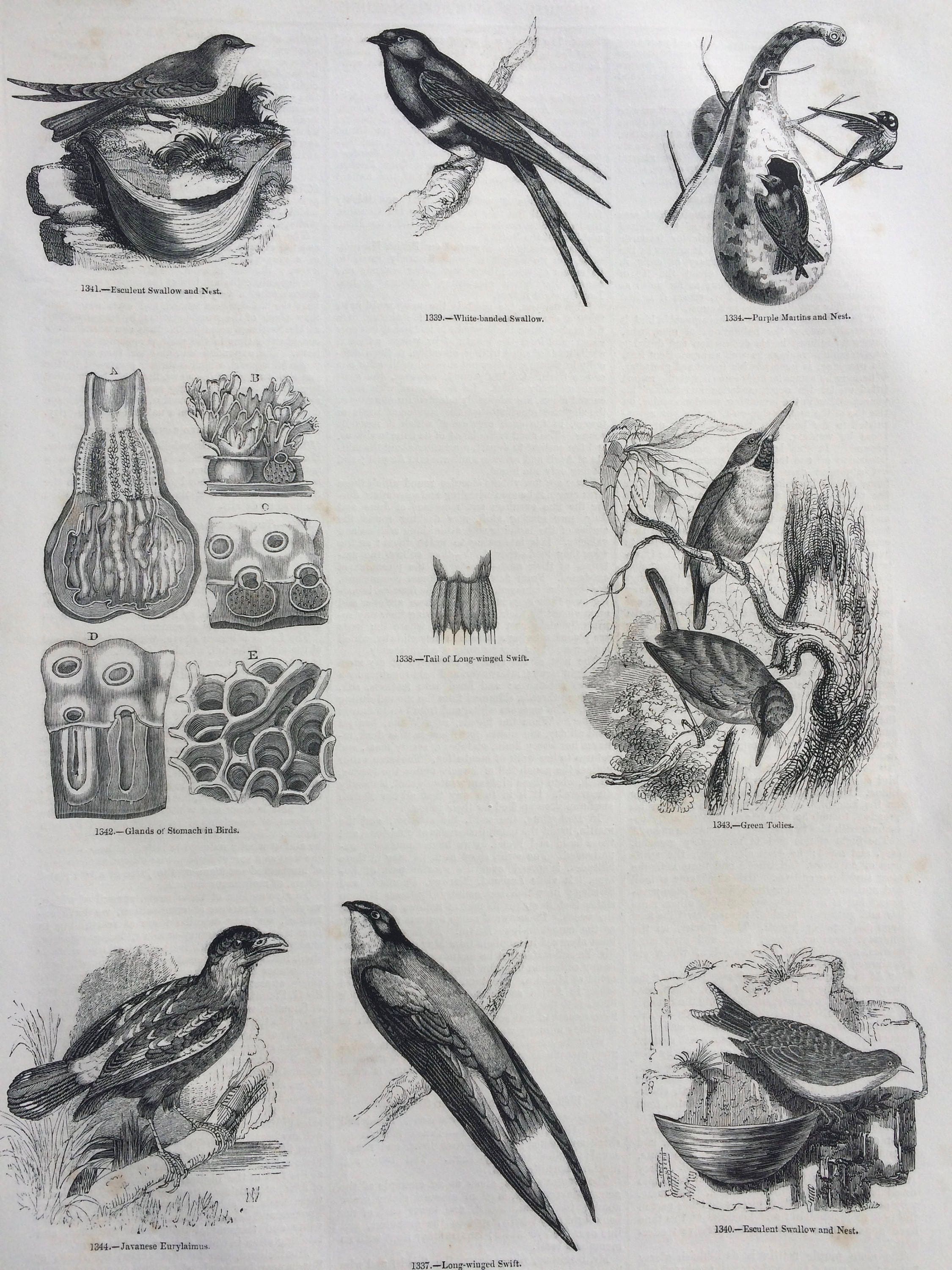This detailed black-and-white poster, set in a horizontal rectangle format, features a variety of bird illustrations accompanied by small black text. In the upper left corner, there are two birds, one perched on a platform and another possibly beneath it, both involved in nest-building. To the right, a long-tailed bird is seated on a branch facing left, followed by another nest scene on tree branches with a bird perched nearby and another in the nest. Below these, in the middle left section, several intricate illustrations possibly depicting nest parts or structural details are visible, followed by a small drawing in the center which includes intersecting lines and five oblong shapes. To the right of this, a person wearing a hat appears to have a bird on their arm. At the bottom, the sequence continues with three separate bird images: one on a branch, another on a branch looking up, and the last one interacting with a nest against a rocky backdrop. Additional details include six illustrations at the bottom, where birds are depicted either perching or nesting, each labeled with descriptive text.